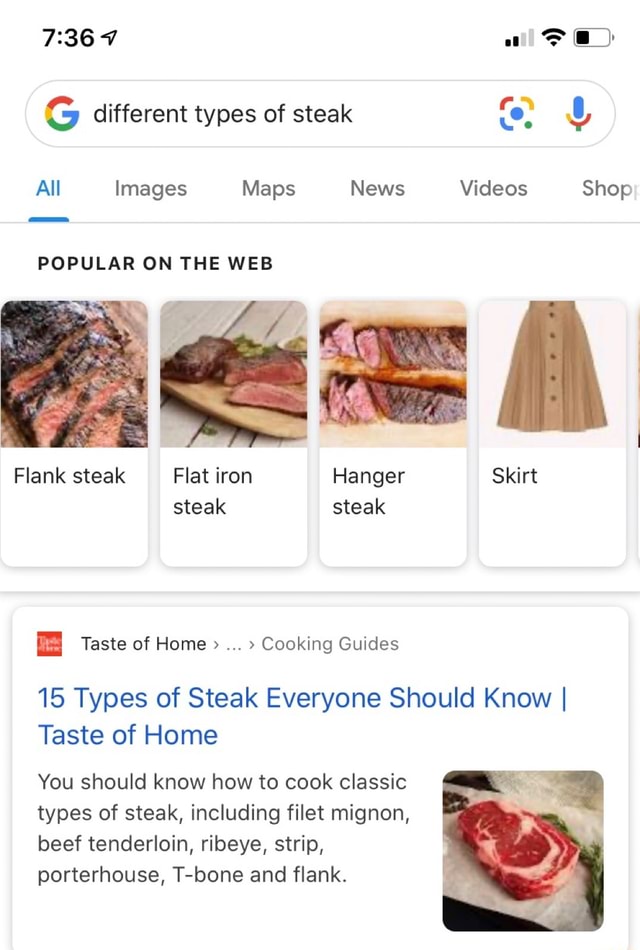A mobile phone screenshot displays a Google search results page at 7:36. The search query entered is "different types of steaks." The top result showcases images and text, with pictures of various steak cuts named flank steak, flat iron steak, and hanger steak. Interestingly, the fourth item, labeled "skirt," depicts an actual beige-colored skirt rather than a meat cut. The first article listed is from Taste of Home, titled "15 Types of Steak Everyone Should Know," highlighted in blue font. Beneath the title, a brief description spans four lines of text. To the right of the text snippet, there is a photo of a steak. The article mentions classic steak types, such as filet mignon, beef tenderloin, rib eye, strip, porterhouse, T-bone, and flank.